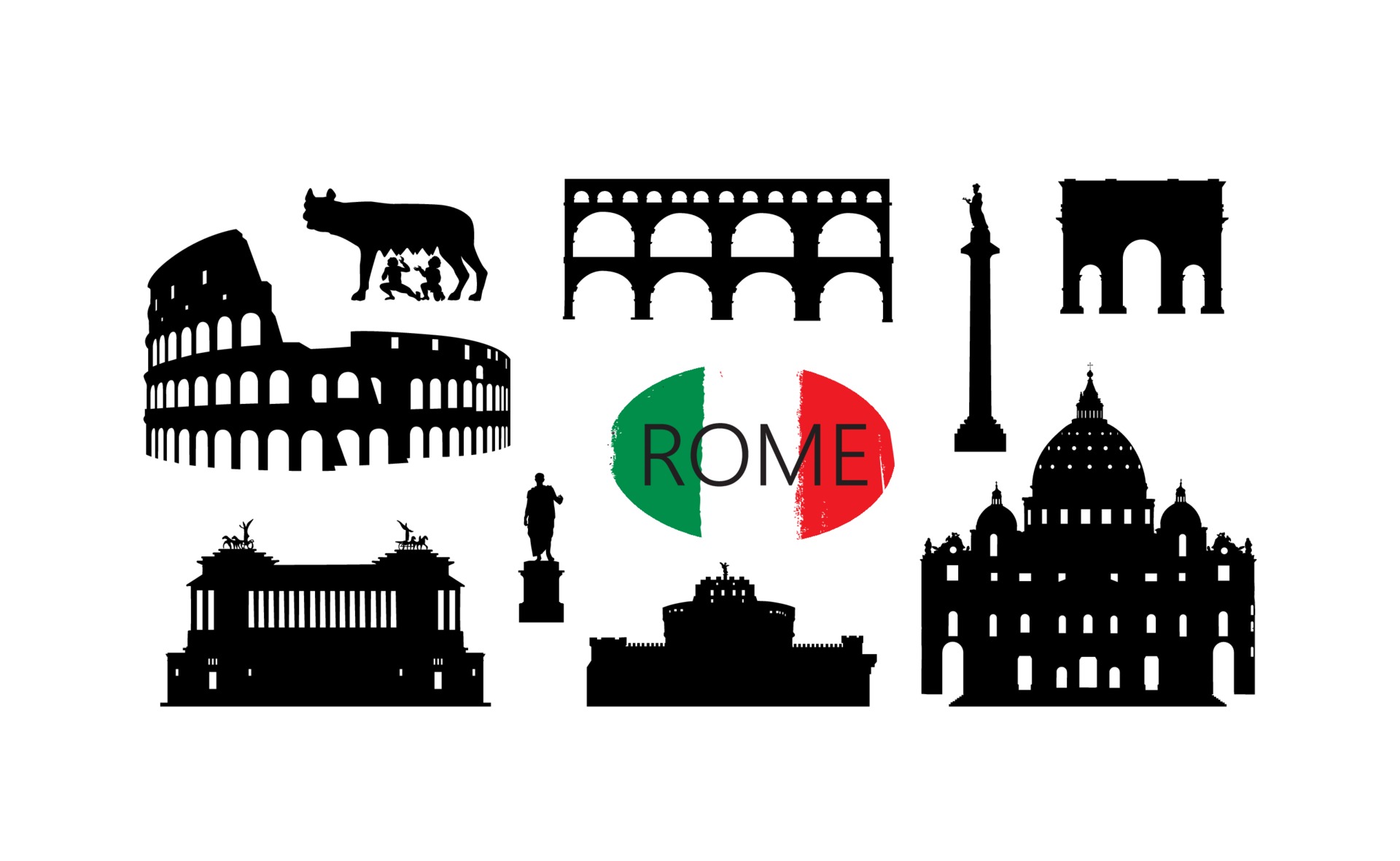The image features silhouettes of various iconic Roman structures set against a white background, designed as a promotional piece for Rome. At the center, an oval encloses the Italian flag with "Rome" written in black script. Surrounding this focal point are nine famous landmarks of Rome, depicted in silhouette. These include the ancient Roman Colosseum and a distinct aqueduct with triple arches. There's also an arch which could be the Arch of Constantine, the Vatican, and the Vatican Square. Additionally, the silhouettes feature what appears to be a statue with two kneeling figures, reminiscent of the Capitoline Wolf, and an obelisk similar to those found in St. Peter's Square. The silhouettes also showcase other statues and architectural wonders, encapsulating a sense of Rome’s historic grandeur.